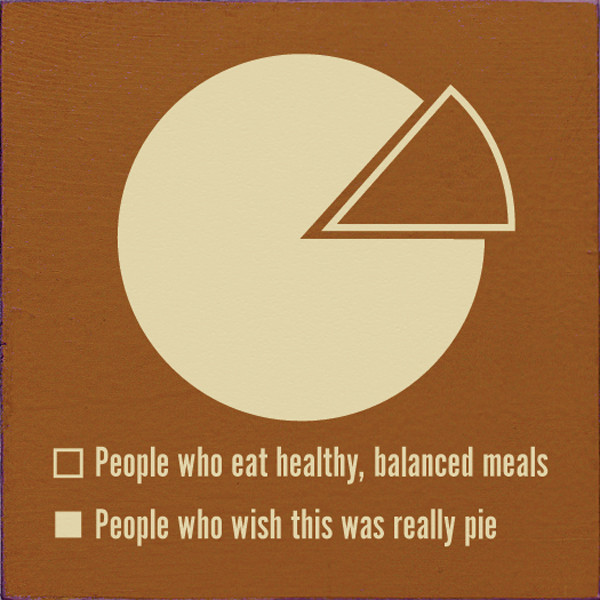The image features a large white pie chart against a solid mocha brown background. The background is square, and at the center of the image is a cream-colored circular shape representing the pie chart. The upper right section of this circle has a triangular slice cut out, mimicking the appearance of a Pac-Man. The cut-out triangle is outlined in the same cream color, but the interior of this outline remains the mocha brown, blending seamlessly with the background. Beneath the pie chart, two bullet points are positioned in a vertical layout. The first bullet point is a brown square with a white outline and white text that reads "People who eat healthy, balanced meals." Below it, a filled white square contains the text "People who wish this was really pie" in brown, matching the background color. This clean and concise visualization juxtaposes humorous and practical perspectives on healthy eating.